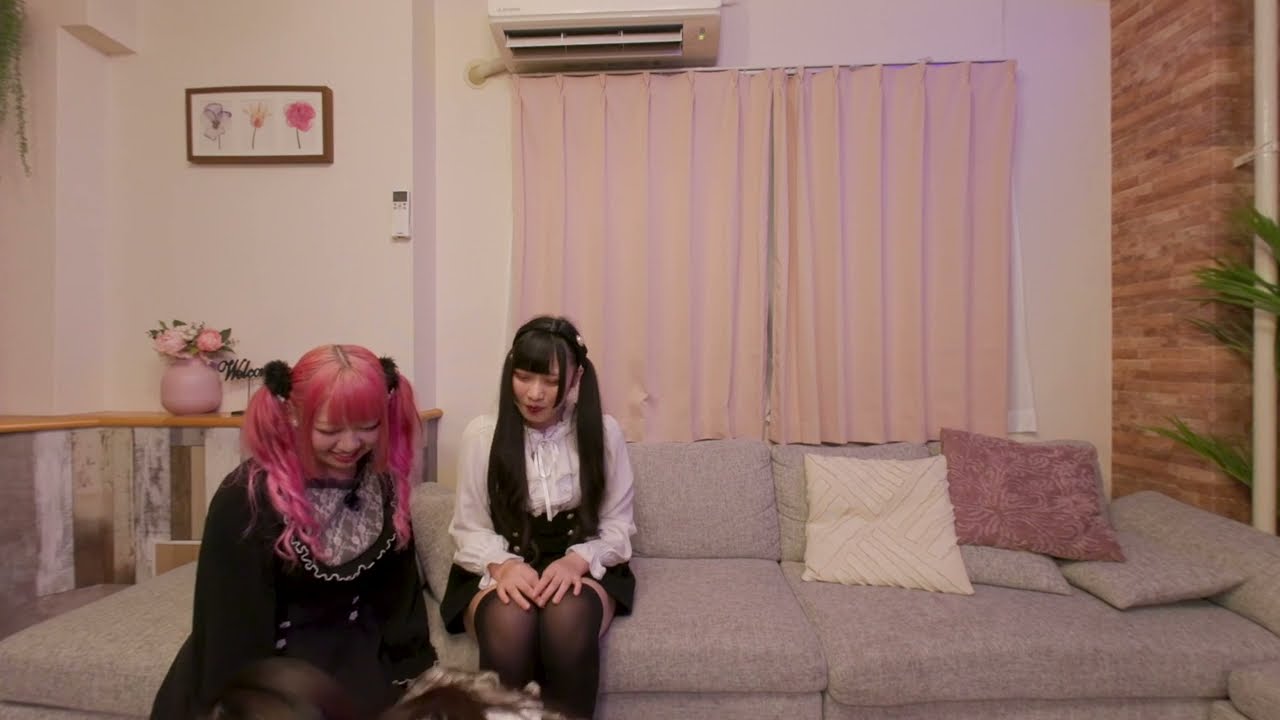The photograph captures a cozy indoor living room scene featuring two young Asian women with distinct alternative fashion style, possibly goth. They sit side by side on the left section of a gray L-shaped sectional sofa, which faces an off-white wall adorned with a picture of three flowers in a white background with a brown frame. Above them, a mounted heating and cooling unit is visible. The prominent feature behind them is a large window with light pink, salmon-colored curtains drawn shut, complemented by a pink vase with flowers on a chair rail beneath it. 

The woman on the far left has striking long pink hair styled in wavy pigtails with black scrunchies. She wears a black top paired with black stockings and has a cheerful expression as she looks slightly downward. To her right sits the second woman, with sleek, long black hair featuring bangs. She is dressed in a white blouse, black skirt, and thigh-high black stockings, and her gaze is similarly directed downward. Decorative pillows—one pink and one white—adorn the couch, and the scene is subtly framed by green foliage from a plant on the right. The overall atmosphere suggests they are focused on something out of frame, perhaps on a coffee table in front of them.